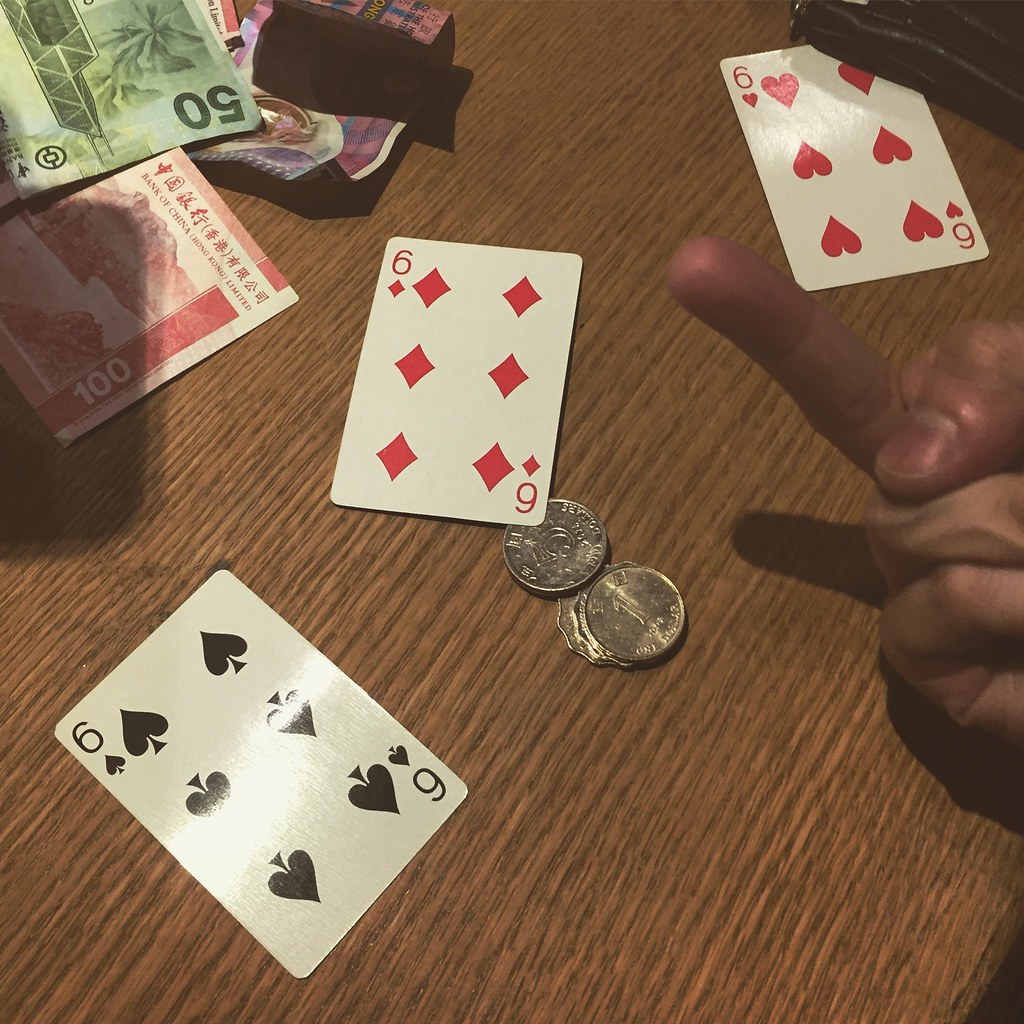In this intriguing photograph, three playing cards – a six of spades, a six of diamonds, and a six of hearts – are neatly arranged on a textured wooden table. The cards are white, with black numerals and pips for the six of spades, and red numerals and pips for the six of hearts and six of diamonds. A conspicuous hand is gesturing forward, its middle finger pointed up in a noticeable stance. Below the six of diamonds, three coins are meticulously placed. Above these coins, an assortment of foreign currency adds a splash of color and intrigue to the composition. A green bill marked with '50', a red bill marked with '100', and a crinkled purple bill are prominently displayed, hinting at diverse origins. The wooden table's prominent grain enhances the rustic aesthetic of the scene.